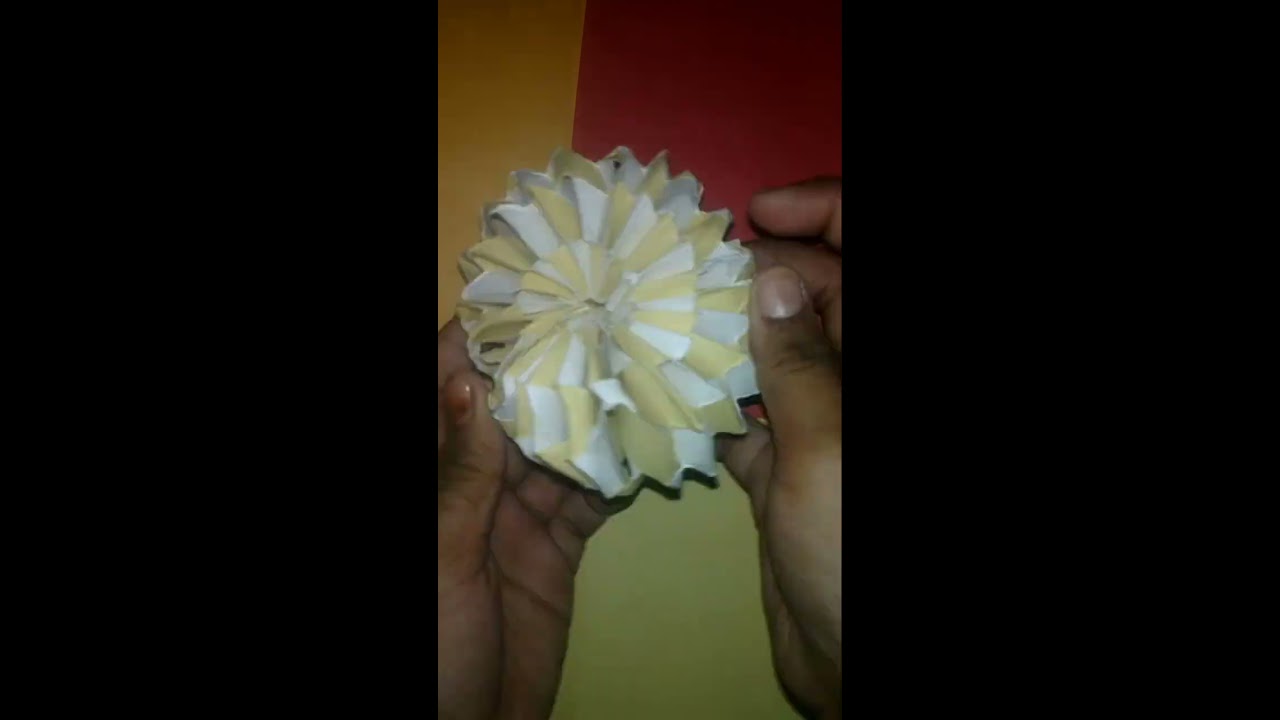The image is divided into three parts, with the left and right sides being completely black. The central section showcases an intricately folded, tan and white paper flower held delicately by a person's hands. The flower, resembling an origami sculpture, features several circular rows with alternating patterns that evoke the look of roofing material. The person holding the flower uses the tips of their fingers and thumbs, with a hint of red-orange nail polish on the left thumb and none on the right hand, which appears a bit dirty or possibly paint-stained. Behind the flower, the background is divided into a red, mustard-yellow, and olive green panel. The flower is positioned closer to the top of the central section, approximately three-quarters of the way up, while the hands rest underneath, framing the artwork. The detailed contrast and positioning within the frame highlight the delicate craftsmanship of the flower against the vibrant yet muted backdrop.